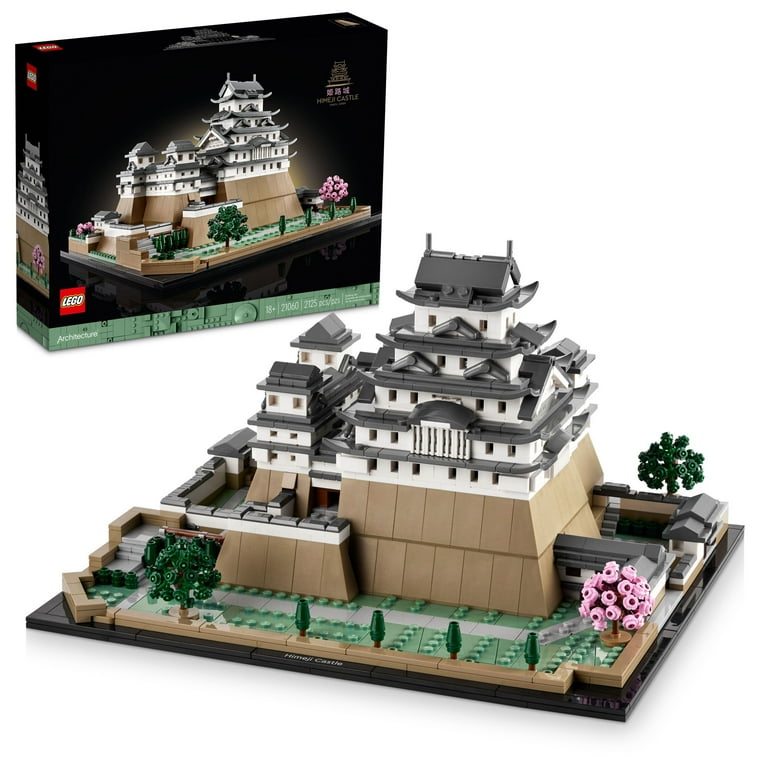This detailed LEGO set features the iconic Himeji Castle, a Japanese architectural marvel. The completed structure sits atop a hill with a brown base, adorned with green pieces representing grass and several small trees, including cherry blossom trees. The castle itself stands at around five stories tall, showcasing a striking contrast of white and gray walls atop its robust wooden-colored foundation. The LEGO set's packaging appears in the top left corner of the image, featuring a black background with a detailed picture of the completed castle, accompanied by Japanese text and the LEGO brand logo. The Himeji Castle sits on a black-bordered platform with its name printed clearly, and the set comprises 2,125 pieces, intended for builders aged 18 and above. The intricacies of this set include windows, staircases, boundary walls, and a lush garden area, making it a masterpiece of Japanese architectural LEGO design.